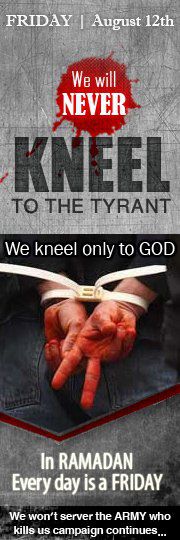The narrow vertical rectangular image, resembling a poster, features a predominantly light gray background with various text sections in bold, contrasting colors. At the top, in white lettering, it announces "Friday, August 12th." Below this, a striking red blotch, reminiscent of a blood drop, bears the text "we will NEVER," with "NEVER" in very large print. Beneath this, the words "kneel to the tyrant" are displayed in dark gray letters on the light gray background. A black section follows, showing two hands tied together and marked with blood. Above the hands, in white letters, it declares "we kneel only to God." Below this statement, larger white letters proclaim "in Ramadan, every day is a Friday." The image uses colors like gray, white, red, dark gray, black, tan, pink, and orange, and suggests themes of resistance and religious devotion. The entire composition emphasizes solidarity and defiance against oppression.